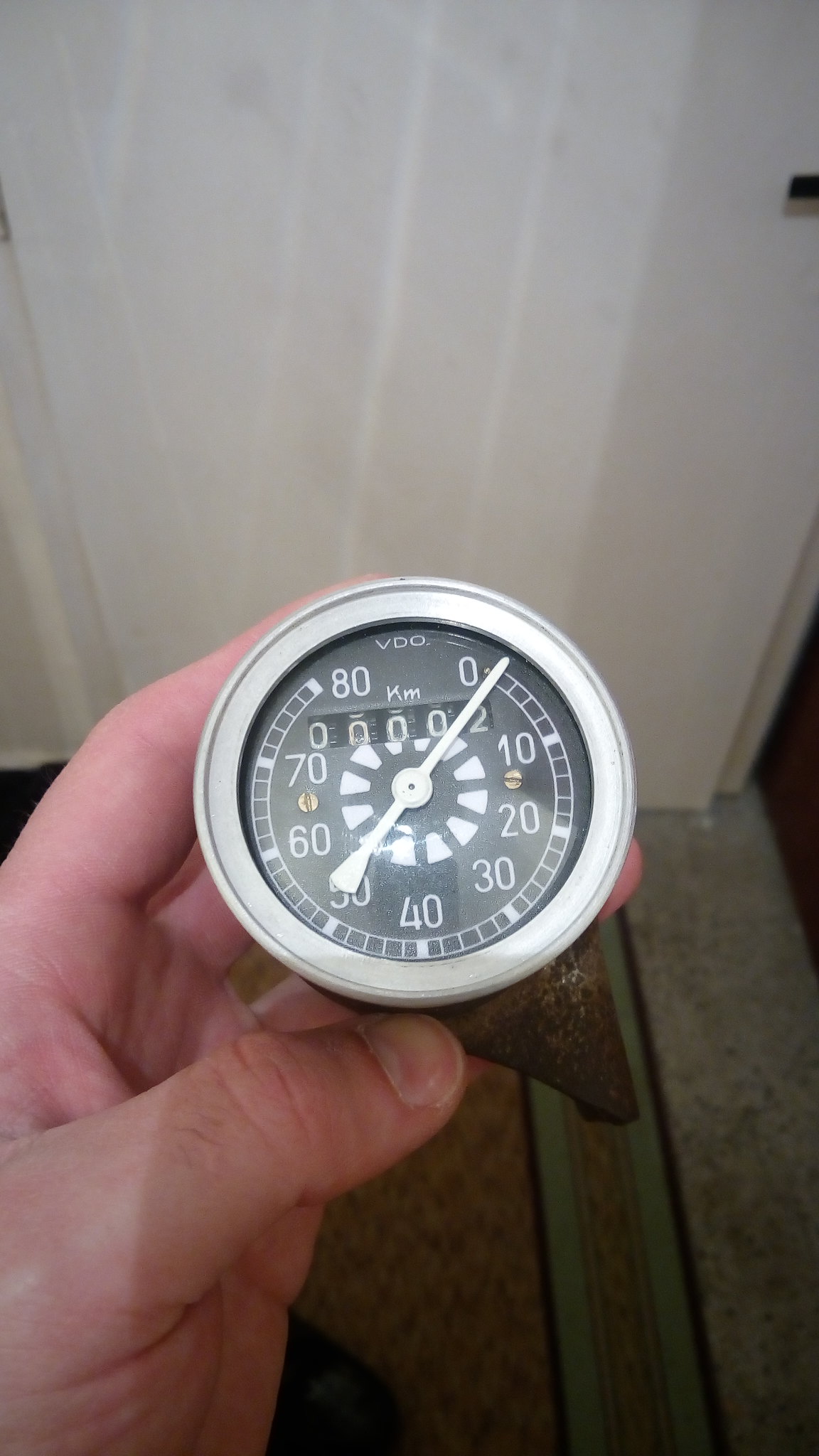The image depicts a close-up photograph of a hand holding a small, circular speedometer positioned directly in the center. The speedometer features a white outer rim, a black face, and white indicators and numerals, ranging from 0 to 80 kilometers per hour. The brand "VDO" is prominently displayed on the gauge, followed by the abbreviation "KM" for kilometers. The hand, located towards the bottom left of the frame, firmly grasps the device. The setting appears to be an indoor room with a gray floor and a white wall in the background, providing a neutral backdrop that highlights the contrasting black and white colors of the speedometer. The image is an overhead view, capturing the person's perspective as they look down at the speedometer in their hand.